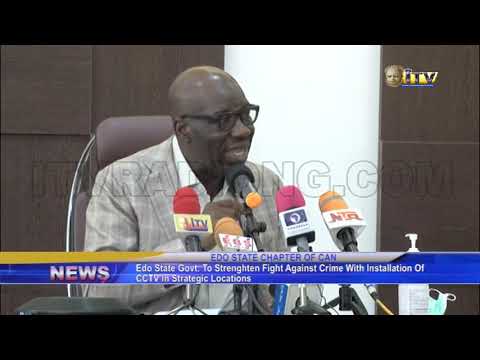The image is a screenshot of a news broadcast, possibly captured from a TV, online production, or a live feed. It shows a press conference featuring an African American man speaking into multiple microphones. The headline at the bottom of the screen reads, "EDO state government to strengthen fight against crime with installation of CCTV in strategic locations." Above this banner, the text "EDO State Chapter of CAN" is displayed. The man, dressed in a light gray suit jacket and white button-down shirt, is seated in a brown office chair with a silver edge. He wears black-framed glasses and is positioned against a background of large brown soundproof or sound panel tiles, with a small section of a white pillar visible to his right. In the upper right corner of the screen, there is a logo for ITV. Additionally, there is a watermark on the image that reads "ITV RAND ONG.com." The overall shot includes a blue and yellow bar designating the news section with the word "NEWS" in red text.